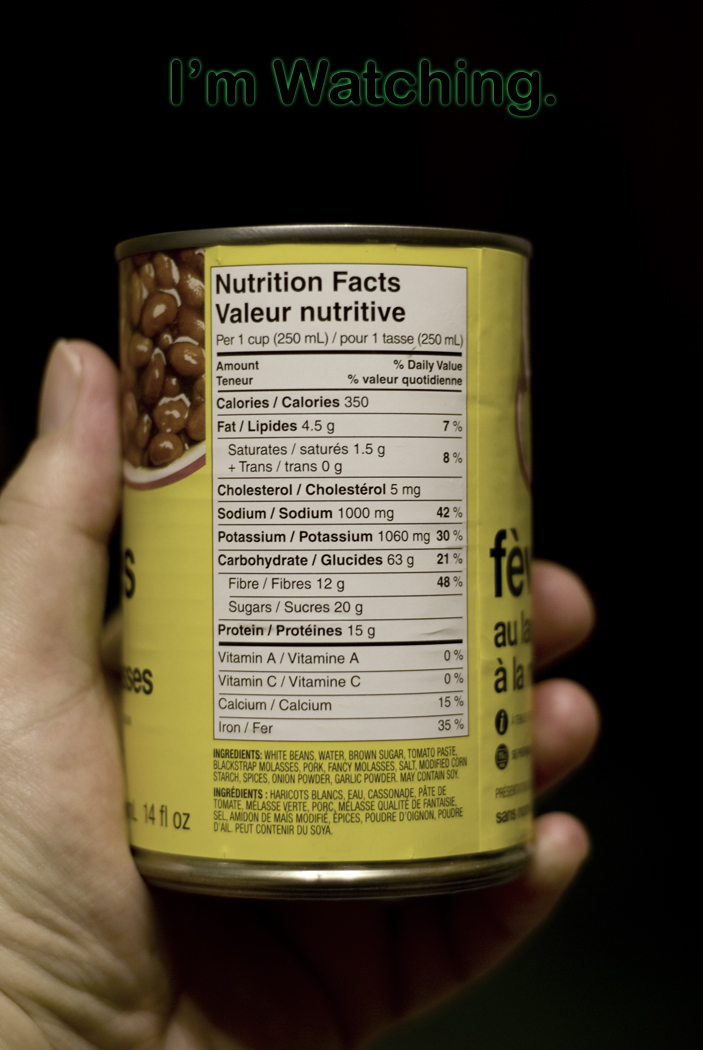In the photograph, the highlighted text at the top of the screen reads "I'm watching." Displayed in black text on a green background, this caption catches one's eye. The focal point of the image is a Caucasian hand holding a 14-ounce can of beans. The can prominently displays a picture of the beans it contains. The side of the can facing the viewer reveals the nutrition facts and a list of ingredients written in black text on a white background. On the right-hand side of the screen, the letters "FE," and underneath them, the letter "U" can be seen, though their context remains unclear.